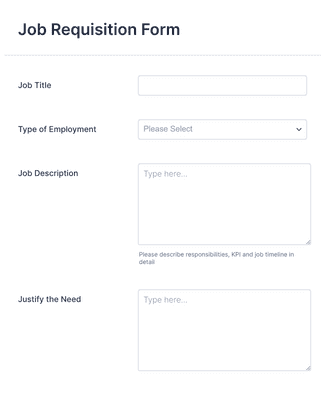The image depicts a Job Requisition Form set against a white background. In the top left corner, the title "Job Requisition Form" is displayed in black text. Below the title, a grey horizontal line stretches across the form. On the left side, smaller black font labels are present. The first label reads "Job Title," followed by a white space designated for input. Below this, the label "Type of Employment" is accompanied by a drop-down box with the placeholder text "Please select." 

Further down, the label "Job Description" appears, followed by another input field with the prompt "Type here," which is currently empty. Beneath this input field, in grey text, it instructs, "Please describe responsibilities, KPI, and job timeline in detail." The subsequent line contains the label "Justify the Need" with a corresponding input field labeled "Type here," which is also vacant.

Overall, the form is structured and organized but entirely unfilled, waiting for input.